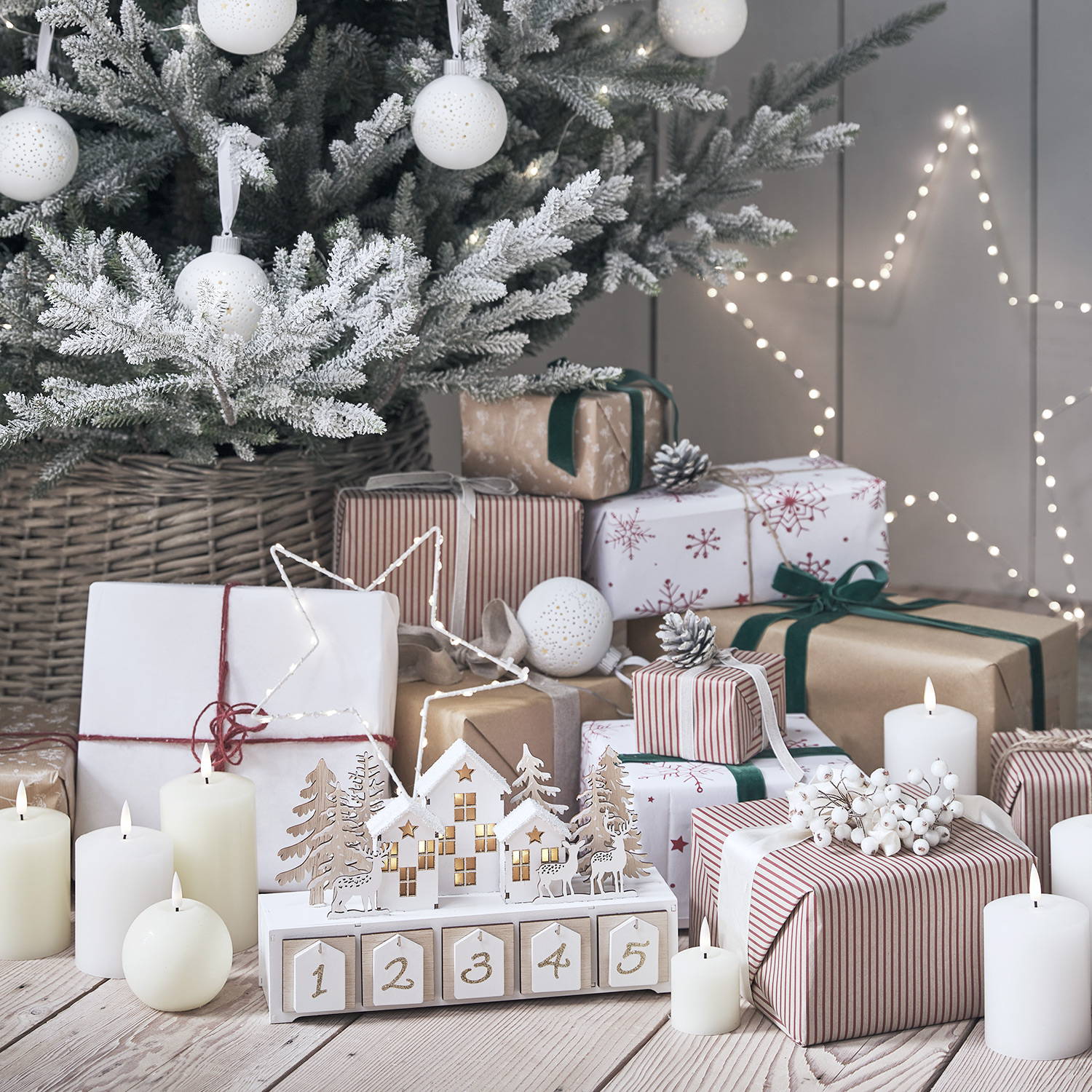This image captures a festive Christmas scene dominated by whites and browns. At the forefront stands a Christmas tree, either naturally white or spray-painted, nestled in a gray wicker basket. Its branches, some frosted and possibly green underneath, are adorned with numerous white, circular ornaments. Behind the tree is a vertical wood wall painted gray, featuring a lit white star made of dotted lights in the upper right-hand corner. The ground beneath the tree is piled high with a variety of presents, some wrapped in white with brownish ribbons, others in brown and white stripes with white ribbons, and even some with red and white stripes. Scattered among the gifts are several lit candles, both cylindrical and circular. Additionally, a charming wooden Christmas scene sits upfront, complete with reindeer, a house, trees, and five small drawers labeled 1 through 5, likely part of an advent calendar or similar festive activity. The overall ambiance of the photo is warm and inviting, with a refined color palette that emphasizes the beauty of a minimalist Christmas décor.